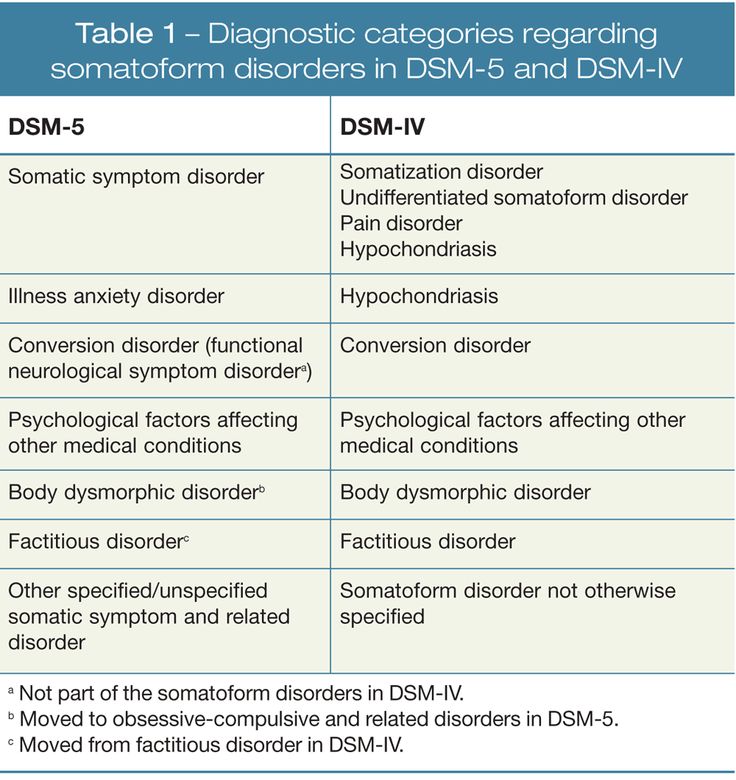**Table 1: Diagnostic Categories Regarding Somatoform Disorders in DSM-5 and DSM-4**

This table illustrates the evolution of diagnostic categories for somatoform disorders between DSM-5 and DSM-4. On the left, DSM-5 introduces updated classification criteria and terminologies, including Somatic Symptom Disorder, Illness Anxiety Disorder, Conversion Disorder, Psychological Factors Affecting Other Medical Conditions, Body Dysmorphic Disorder, Factitious Disorder, among others. On the right, DSM-4 lists the previous classifications: Somatization Disorder, Undifferentiated Somatoform Disorder, Pain Disorder, Hypochondriasis, Conversion Disorder, Body Dysmorphic Disorder, and Factitious Disorder. Notable differences include the consolidation and redefinition of categories, reflecting changes in diagnostic practices and clinical approaches to treating these disorders.